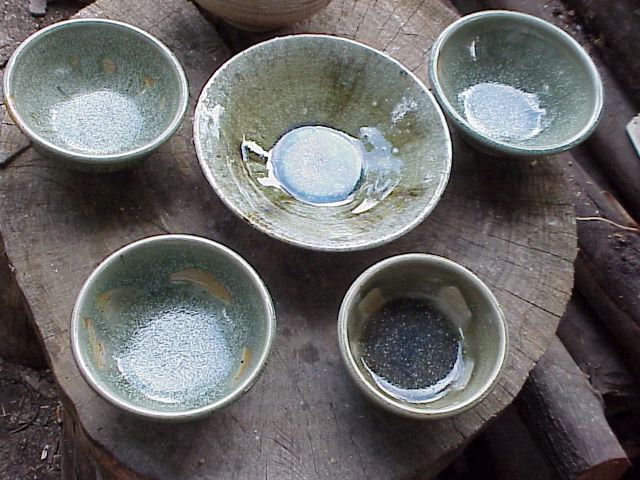The photograph, captured in vivid color, displays a series of handmade ceramic bowls arranged on an aged, light-gray tree stump. The stump, with its flat, weathered surface, serves as a rustic pedestal for six bowls, organized with the largest at the center and five evenly placed around it. This center bowl, more flat and decorative, showcases bands of dark green, light green, and brown, exhibiting a high degree of reflectiveness under the sunlight. The surrounding bowls vary in size, shape, and color; they range from aqua teal to mixed sage green and brown, with some displaying speckled appearances. To the right of the tree stump, logs and branches rest on a dirt-covered ground, adding to the natural outdoor setting of the image.